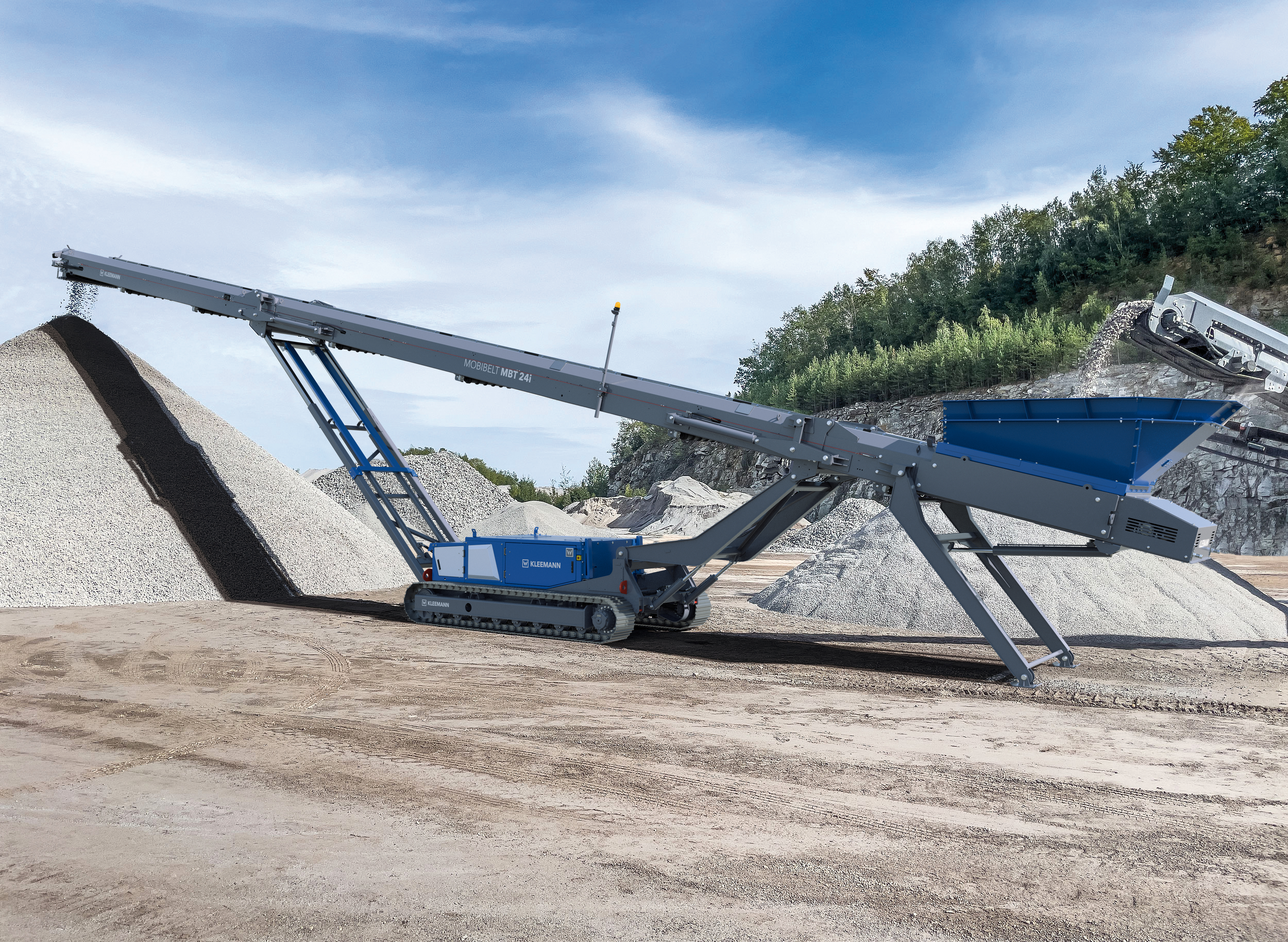The photograph showcases a large, formidable construction machine situated in what appears to be a quarry. The machine is mounted on tank-like treads, displaying a blend of blue and grey hues across its robust frame. Dominating the scene is an extended conveyor belt structure that looms over the machine, stretching from the right side of the image to the left. Gravel is being fed onto this belt by another conveyor, and it travels along the length of the belt before spilling out onto a high, triangular-shaped pile of gravel. Surrounding this principal pile are multiple similarly sized mounds of gravel, adding to the rugged, industrial atmosphere. The landscape, composed of dirt and sediment, underscores the machine's function and the intense, ongoing extraction and processing activities typical of a quarry.